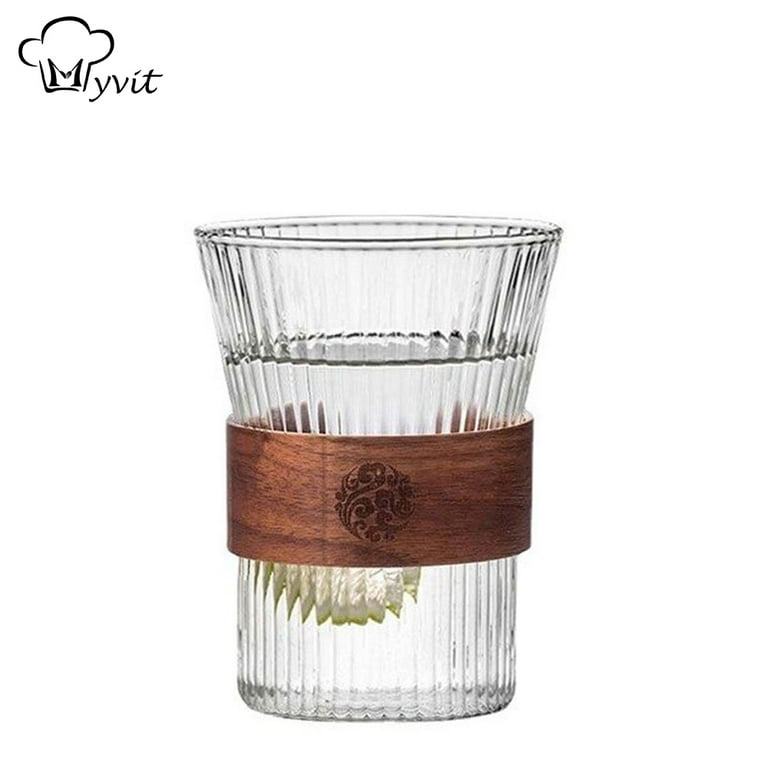The image features a small, decorative drinking glass, commonly seen in the Middle East for tea. The glass is clear, with ridged, fluted vertical lines from the base to the top, where it flares out slightly, forming a delicate V-shape. A distinctive mahogany-colored wooden band encircles the middle of the glass, adorned with an intricately etched floral or paisley pattern. Inside the glass, there appears to be a thin slice of lime amidst some clear liquid, likely water or a translucent beverage, indicating it's filled nearly to the top. In the upper left corner of the image, set against a stark white background, is a black-and-white outline of a chef's hat with an 'M' on it, accompanied by the word 'MYVIT' in a mix of regular and cursive script. The overall design is both simple and elegant, combining traditional craftsmanship with modern aesthetics.